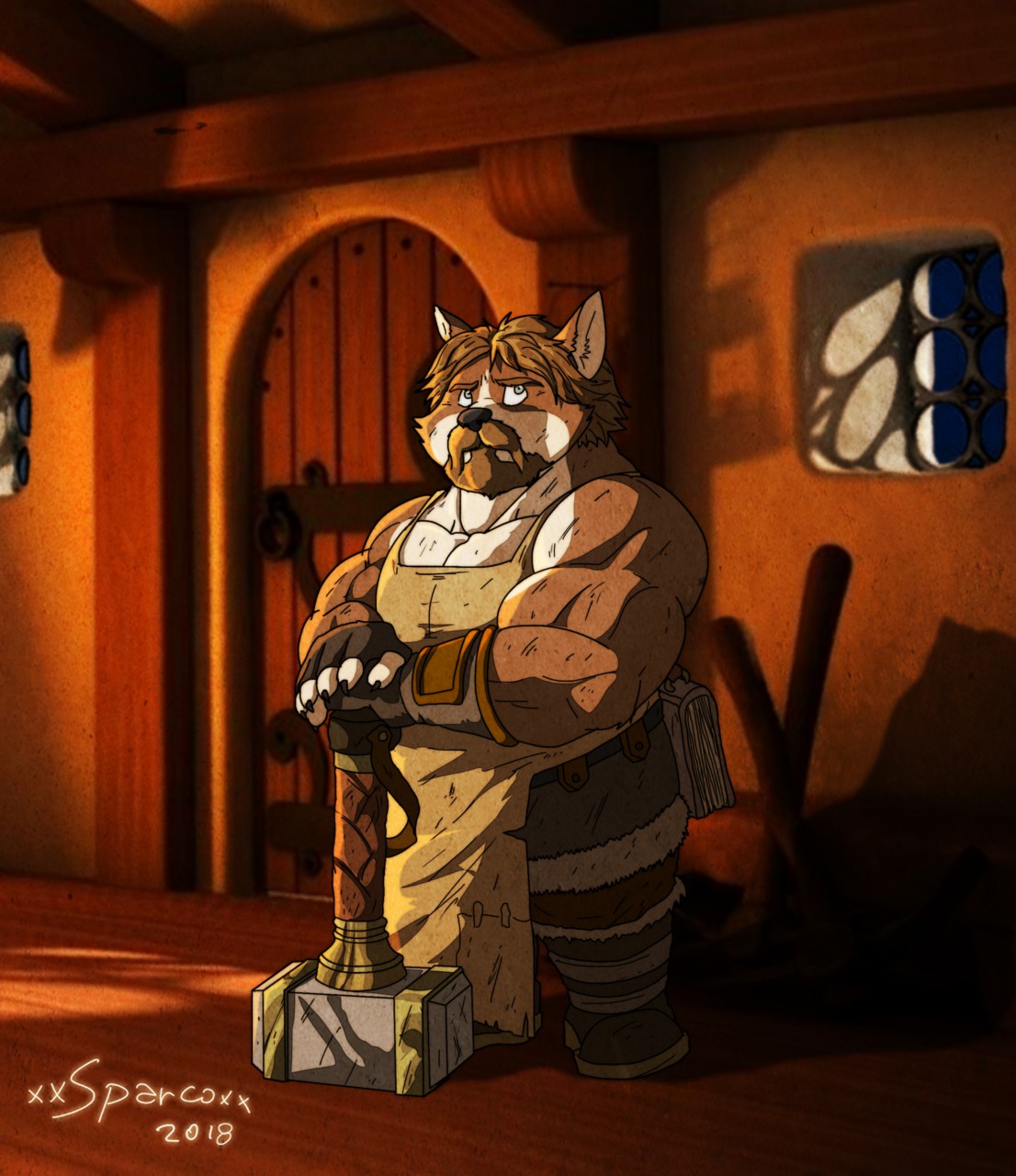The image depicts a cartoon-like character, a burly anthropomorphic dog standing upright, resembling a humanoid figure. This dog-man, with distinct canine features like a snout and dog ears, appears exceedingly muscular with comically large biceps flexed. Shaggy brown hair frames his face, complementing his tan fur and a beard. He dons what looks like an apron, akin to a smithy's outfit, in various shades of brown, akin to a tan Santa suit, accentuated with a heavy belt.

His stance is assertive, leaning slightly to the side while gripping an imposing hammer that resembles Thor's Mjölnir. The hammer's handle is brown with gold accents, and the head is grounded, showcasing his immense strength. His blue eyes gaze off to the side, suggesting a contemplative or dismissive mood.

The setting hints at a medieval blacksmith's workshop or a rustic tavern, featuring reddish-brown walls, wooden support columns, a stout wooden door, and a metal-barred window. Details like a gray stand and possible telescope-like object with a strap add to the scene's character. At the lower left, the artwork is signed "XXSPARCOXX 2018," linking it to the SPARKCON event.